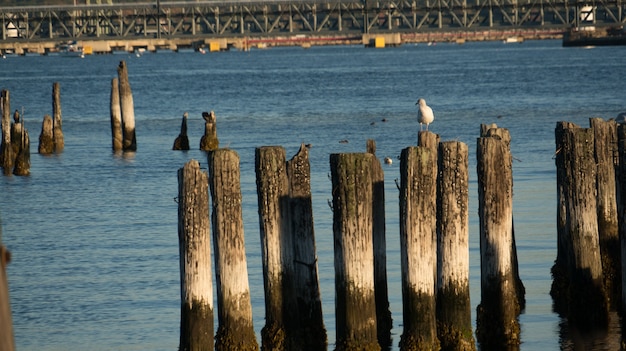The image depicts a serene waterway dominated by expansive blue waters, dotted with rotting wooden posts—remnants of an old, broken dock. At the forefront, a solitary seagull perches on one of the deteriorating wooden beams, its plumage stark against the brown and white of the weathered wood. These posts, appearing wet and cracked at the top, jut out of the calm water, which ripples gently in the image. In the distance, a bridge or possibly a large structure spans across the upper part of the image, adding depth to the background. No boats or people are visible, highlighting the tranquility of the scene. The overall composition, with elements of blue, white, and brown, presents a quiet yet detailed glimpse into this waterscape.